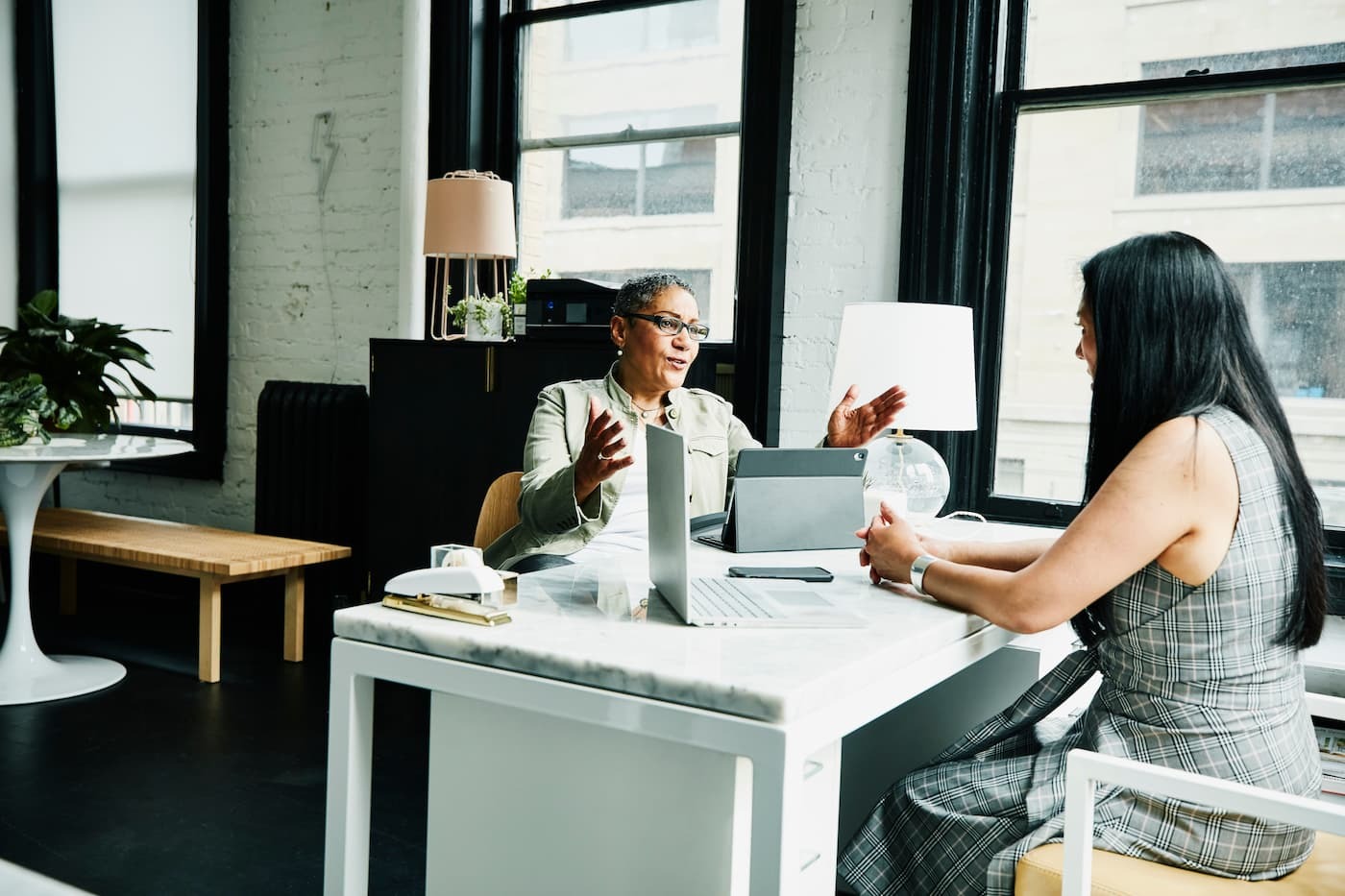In a high-rise office with large windows revealing the neighboring building outside, two women are seated across a white marble-topped desk from each other, engaged in what appears to be a business meeting or an interview. The woman on the viewer's right, seen in profile with her back partially to the camera, has long, shiny black hair and wears a sleeveless black and white plaid dress. Opposite her, the woman with short hair, wearing glasses and a light-colored jacket, has her hair pulled back and is extending both arms forward in an expressive gesture as if making a point. Both women have open electronic devices in front of them—a laptop and a tablet. The desk also features a small white lamp, a phone, and a stapler. In the background, the office has white-painted brick walls, various pieces of furniture including a round white table, a wooden bench, and another lamp, all contributing to the modern and organized ambiance of the space.